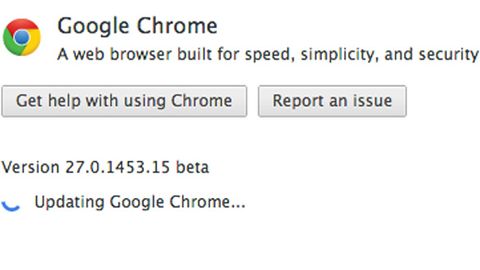**Caption:**

A detailed screenshot of a webpage in landscape orientation featuring the Google Chrome update interface. The page is set against a white background. 

In the upper-left corner, the colorful Google Chrome logo is prominently displayed. To its right, the text "Google Chrome" appears in bold black, followed by the tagline "a web browser built for speed, simplicity, and security."

Below this heading are two wide gray buttons with black text: "Get help with using Chrome" on the left and "Report an issue" on the right. These buttons have a slight drop shadow, adding depth to the otherwise minimal design.

Further down, the text "version 27.0.1453.15 beta" is displayed in black against the white background, indicating the browser version.

Below this version information is a blue semi-circle loading icon next to the text "Updating Google Chrome..." in black, indicating that an update process is underway.

The rest of the image remains blank white, without any borders or additional elements, emphasizing the simplicity and focus of the page’s current purpose.